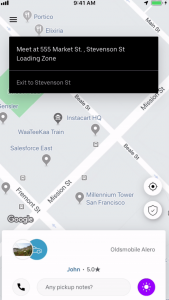The image is a detailed screenshot from a mobile device displaying a street map. The map covers a color palette of different shades of gray and a light gray background, accentuating the white street lines that crisscross across the screen. Various street names are visible, adding to the map's intricacy. Scattered across the map are location icons characterized by black, gray, and white circles, each pointed like a pin at specific locations. In the lower left corner of the screen, there's a black telephone icon. Adjacent to it, on the right side, is a text box with the label "Any pickup notes." Dominating the top portion of the image is a black rectangular box with white text that reads, "Meet at 565 Market Street, Stephenson Street, loading zone."